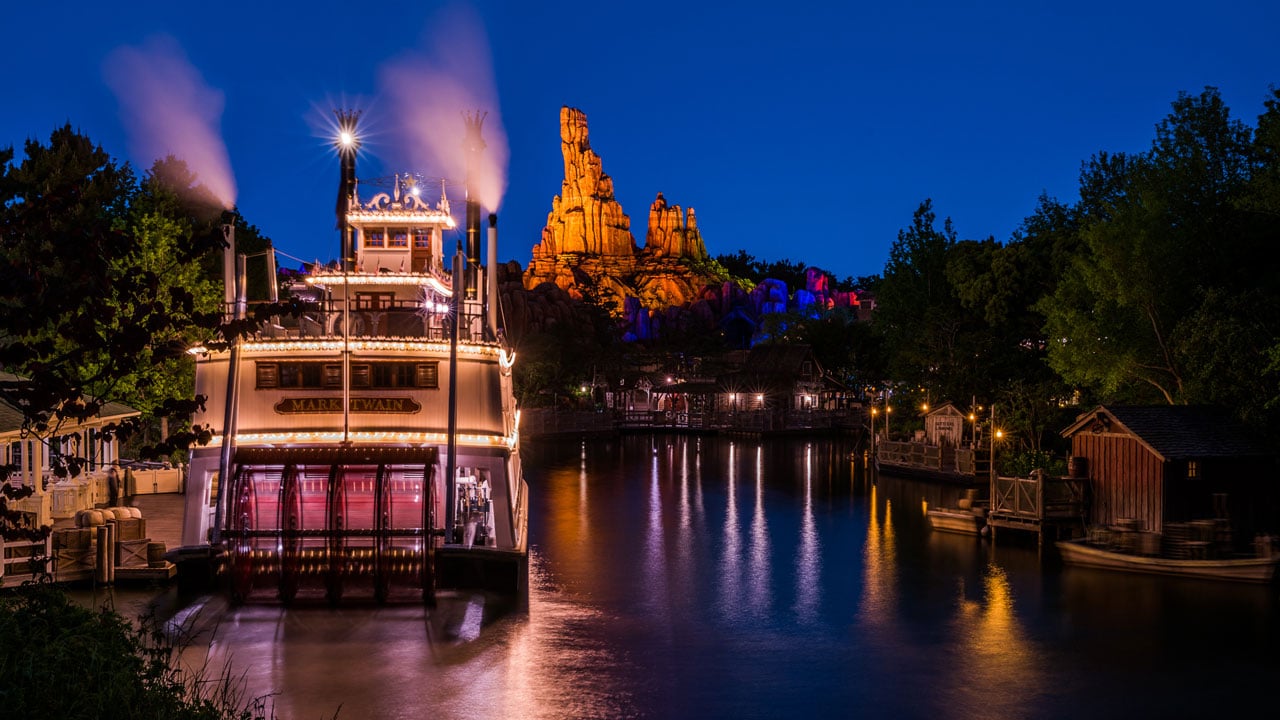The image captures a picturesque nighttime scene reminiscent of a theme park setting, bathed in the serene glow of a dark blue sky. Dominating the left half of the composition is the iconic ferry boat "Mark Twain," a multi-leveled steamboat complete with two prominent smokestacks emitting steam, and large paddle wheels. Strung with lights, this riverboat exudes an inviting ambiance. Reflections from the boat and nearby structures shimmer on the calm water, accentuating the tranquil atmosphere.

To the right, the scene features a charming array of small wooden buildings, including a quaint outhouse-like structure and a more substantial white building, both accompanied by docks and tiny boats. These sit nestled among lush green trees, which create a natural, serene backdrop.

Further back, and central in the frame, stands an impressive, well-lit building, its elegance adding a touch of grandeur to the landscape. The far background reveals a dramatic, naturally-styled rock formation, some parts illuminated with enchanting blue and pink lights, completing the scenic vista. This detailed and idyllic night scene seems perfectly designed to entice visitors, capturing the essence of a magical waterfront destination.